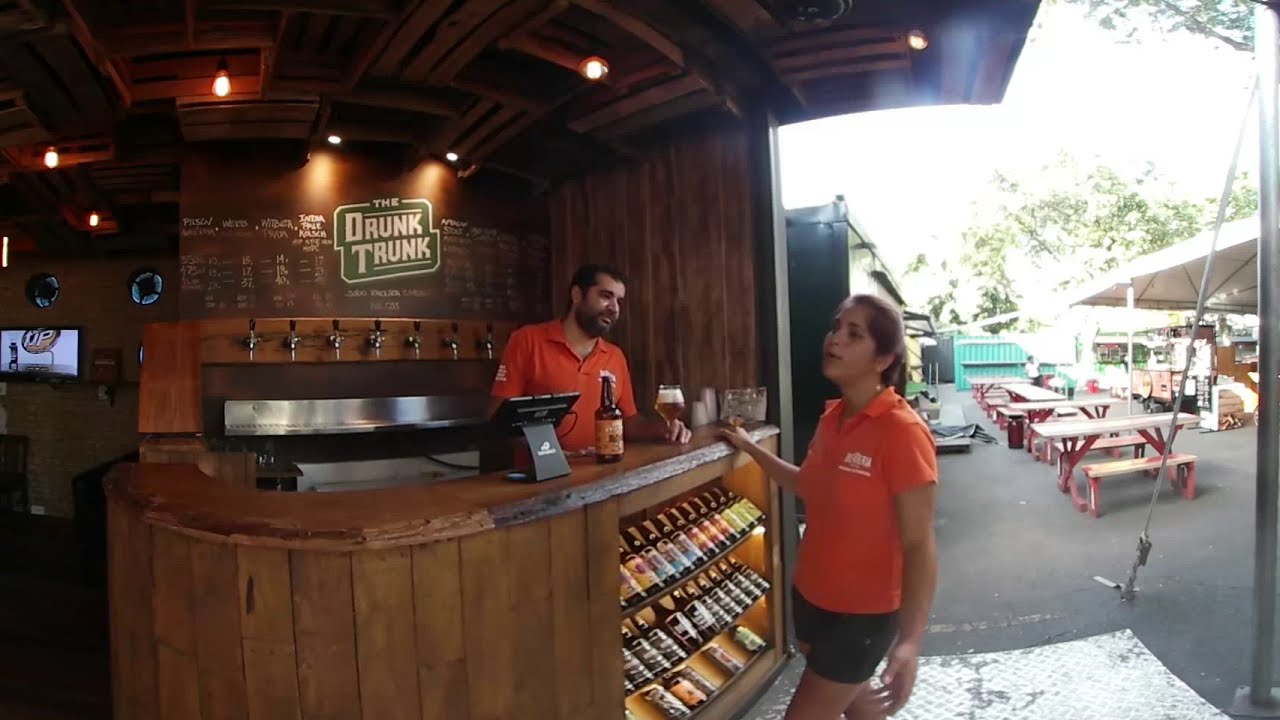The image depicts an outdoor bar stand named "The Drunk Trunk," as identified by a sign in the interior. The bar is constructed of brown wood and features a wooden roof, open to outdoor surroundings. Standing behind the counter is a man with dark hair and features, and he is wearing an orange short-sleeve polo shirt. He appears to be holding a large bottle of alcohol and a foamy, filled glass that resembles a wine or champagne glass. His elbow rests casually on the counter. 

Opposite him, on the other side of the bar, stands a woman dressed in a similar orange short-sleeve polo shirt paired with black shorts. Her long hair is tied back in a pigtail, and she is engaging with the bartender while facing towards the left. 

In the bar setup behind the bartender, there are multiple beer taps lined up on the wall, at least seven in total. Above these taps is a chalkboard with a price list written in white chalk. The bar area also includes a point-of-sale touchscreen and beer cans placed on the counter alongside a cash register. 

To the right, outside the bar area, picnic tables are placed on a black macadam surface, alongside a patio area featuring tables and benches, likely situated on cement or concrete. The backdrop includes glimpses of the sky with glare, some trees, and a pop-up tent sheltering numerous boxes. Additionally, the left side of the image reveals an indoor café area with visible lighting and what appears to be a television in the far corner, suggesting there is covered seating available as well.